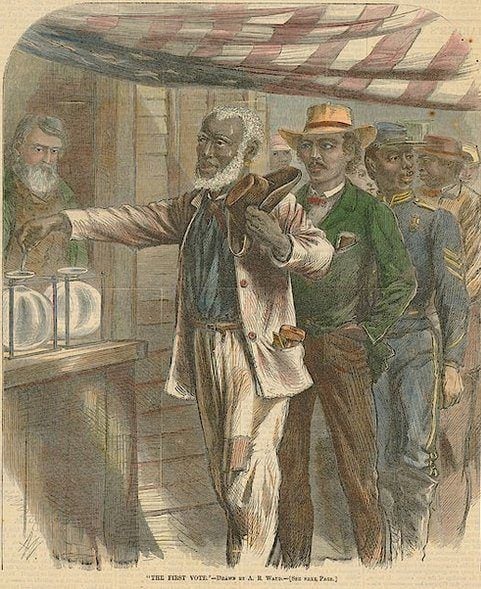In this detailed and emotive illustration, set in an outdoor setting, six men line up in front of a wooden shop with a window open to the inside. Above the scene, an American flag, draped like a banner, adds a patriotic feel to the imagery. A tent with red and yellow stripes provides shade for the men below. The focus is on four African-American men, casting their votes. The first man, notable for his white beard, white shoes, white pants, and holding a hat, is depicted dropping a ballot into a glass jar placed on the window ledge. Another jar sits nearby on the ledge. Behind the jars, through the window, a man with gray hair and wearing a green coat observes the proceedings.

Next to the first voter stands a man in a green suit, yellow cowboy hat, and blue pants. Following him, a third man dressed in a blue soldier's uniform signifies his association with the Northern Army of the Civil War. Detailed and washed-out, the illustration captures the significance of the moment, encapsulated by the inscription at the very bottom, "The First Vote." This poignant artwork vividly narrates a historic event, emphasizing the critical moment of these men casting their ballots, signifying their newly won rights.